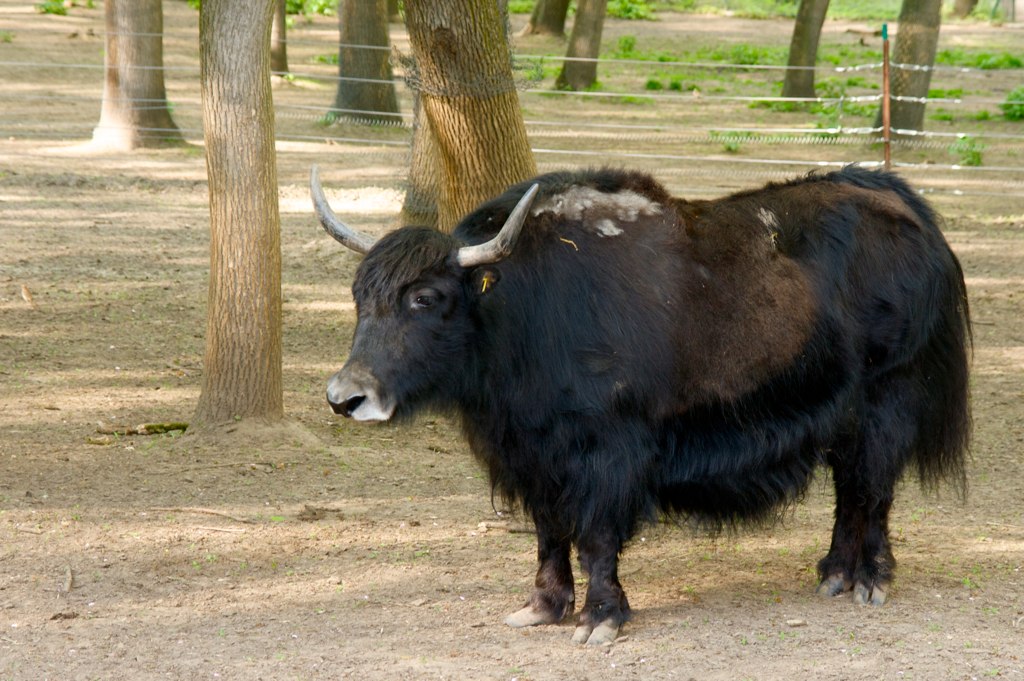This image depicts a large, rugged bovine animal that appears to be a cross between a bull and a bison, or possibly an ox. The creature is predominantly black with shaggy, long fur interspersed with patches of brown, giving it a mottled appearance. Its fur, particularly dense and woolly, almost obscures its relatively short brown legs, making them appear stubby. The animal features a pronounced hump at its shoulders and sports two long, lighter brown horns with black tips extending from the sides of its head. The face is mostly black, with a black nostril and a contrasting white nose, and tufts of longer, darker brown fur on top of its head add to its wild look.

The animal stands in a dirt-floored enclosure, devoid of grass, which has clearly seen heavy trampling. Surrounding the enclosure are metal posts with electrified wires spaced about six inches apart, forming a barrier around the area. Trees are present both within the enclosure and in a neighboring one visible in the background. The branches and tree trunks add a natural element to the otherwise bare, dirt-covered ground. The overall setting suggests a carefully contained environment designed to house and perhaps protect this unique and intriguing creature.